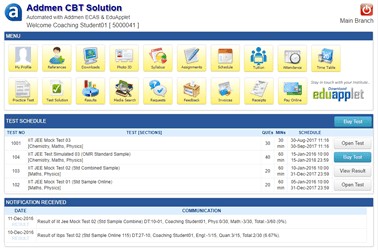This image, taken from a website, features a white background in the top left corner. Adjacent to it, on the right, is a blue circle housing a bolded, lowercase white "A." Below this icon, "Admin CBT Solution" is spelled out in small black capital letters. Underneath, in a slightly larger font, it reads "Automated with Admin CAS and EduApplet." Following this text is a phrase, "Welcome Support Student," with a numeric identifier, "(5000041)," in parentheses.

On the right side of the image, there's a prominent red square containing a power button symbol, with the words "Main Branch" in black lettering below it. A blue border labeled "Menu" is positioned on the left side of the image.

The layout includes several neatly arranged squares with a tan background, displaying various icons and labels such as "camera," "schedule," "profile," etc. Specifically, there are ten squares in the top row and nine in the second row.

To the right of the bottom row, there's a distinctive section with the word "Edu" in green, "APP" in blue, and "LET" in gray. Above this segment, some text is visible, though not clearly legible. Below it, a white border is followed by a blue strip.

To the left of this section, the phrase "Test Schedule" is displayed. On the right, a light blue tab reads "By Test." Below, information is organized into columns: test number on the left, test name to the right of it, followed by a "View Results" button. Additional tabs next to it display further details like schedule dates, duration, and the number of people waiting.

At the bottom, the phrase "Notification Received" is present, accompanied by a date on the left side and corresponding message details on the right side.